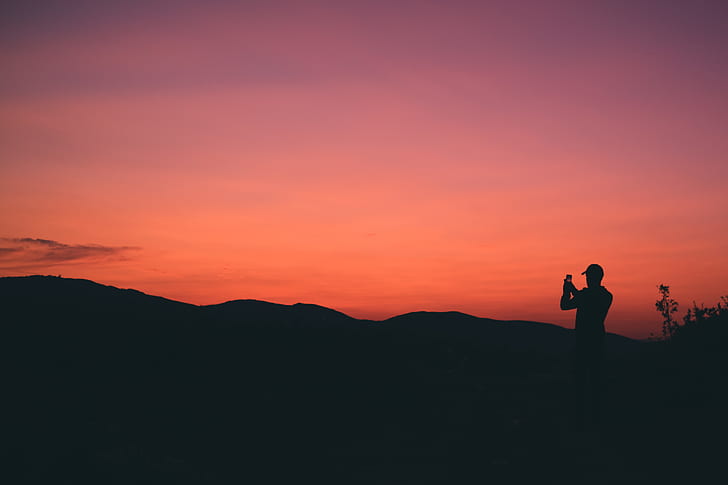In this color landscape photograph, we observe a man silhouetted against a mesmerizing sunset. Situated at the bottom right of the image and visible from head to waist, he appears to be taking a cell phone photo, with his hands raised and the phone centered in his grip. The man, who is wearing a cap with a visor, stands out as a dark silhouette, seamlessly blending into the similarly black silhouette of the smooth, rolling mountain range behind him. The sky transitions from a deep purple at the top to a vivid orange near the horizon, where streaks of vegetation gently emerge in the background. Both the man and the mountain range are prominent against this breathtaking gradient, creating a harmonious balance between the natural and human elements in this scene of photographic realism.